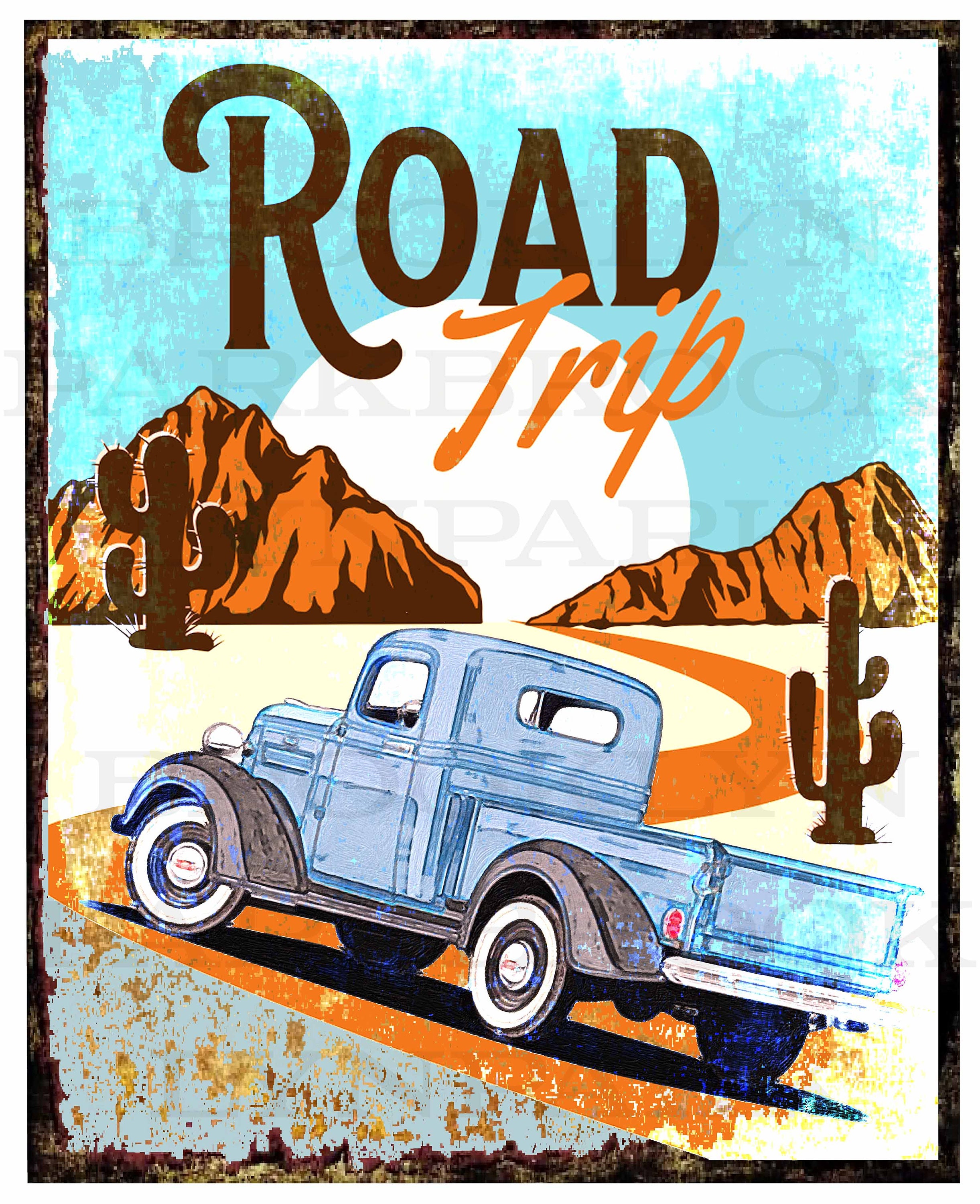This image is a detailed, non-realistic artwork or poster with a vintage, distressed finish depicting a desert road trip scene. The foreground features a light blue, 1940s-era vintage pickup truck with gray wheels and black fenders, driving along a winding, orange road. On either side of the road stand two brown cactuses, a larger one on the left and a smaller one on the right, set against the backdrop of orange and brown mountain ridges which reflect shadows. 

The sky above is a splattered blue, transitioning to a white-hued sun that is slightly covered by these canyons. The words "Road Trip" dominate the image, with "Road" written in a large, brown swirly font and "Trip" in a smaller, orange font that starts beneath the letter 'A'. There's also a faint text in the background, adding to the weathered look, suggesting it might be an advertisement. The setting likely represents the American Southwest, giving a sense of the open road and adventure common to retro desert themes.